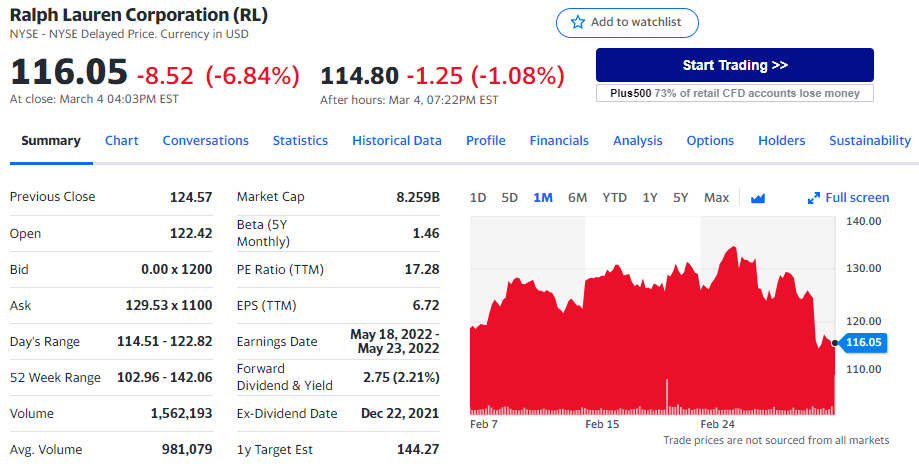This image captures a detailed snapshot of the Ralph Lauren Corporation (RL) stock performance on a trading platform. The stock is shown to be priced at $116.05, reflecting a significant decrease of $8.52, or -6.84%, from its previous value. At market close, the price dipped further to $114.80, marking an additional decline of $1.25 or 1.08%. Below the stock price information, there is a navigational tab displaying various sections such as Summary, Chart, Conversations, Statistics, Historical Data, Profile, Financials, Analysis, Options, Holders, and Sustainability.

In the lower part of the image, a red chart is prominently displayed, visualizing the stock's declining trend over a specific time period. The left side of the chart lists various stock prices, while the right side displays corresponding numerical data points. This detailed image provides a comprehensive view of Ralph Lauren Corporation's stock performance and related financial data.